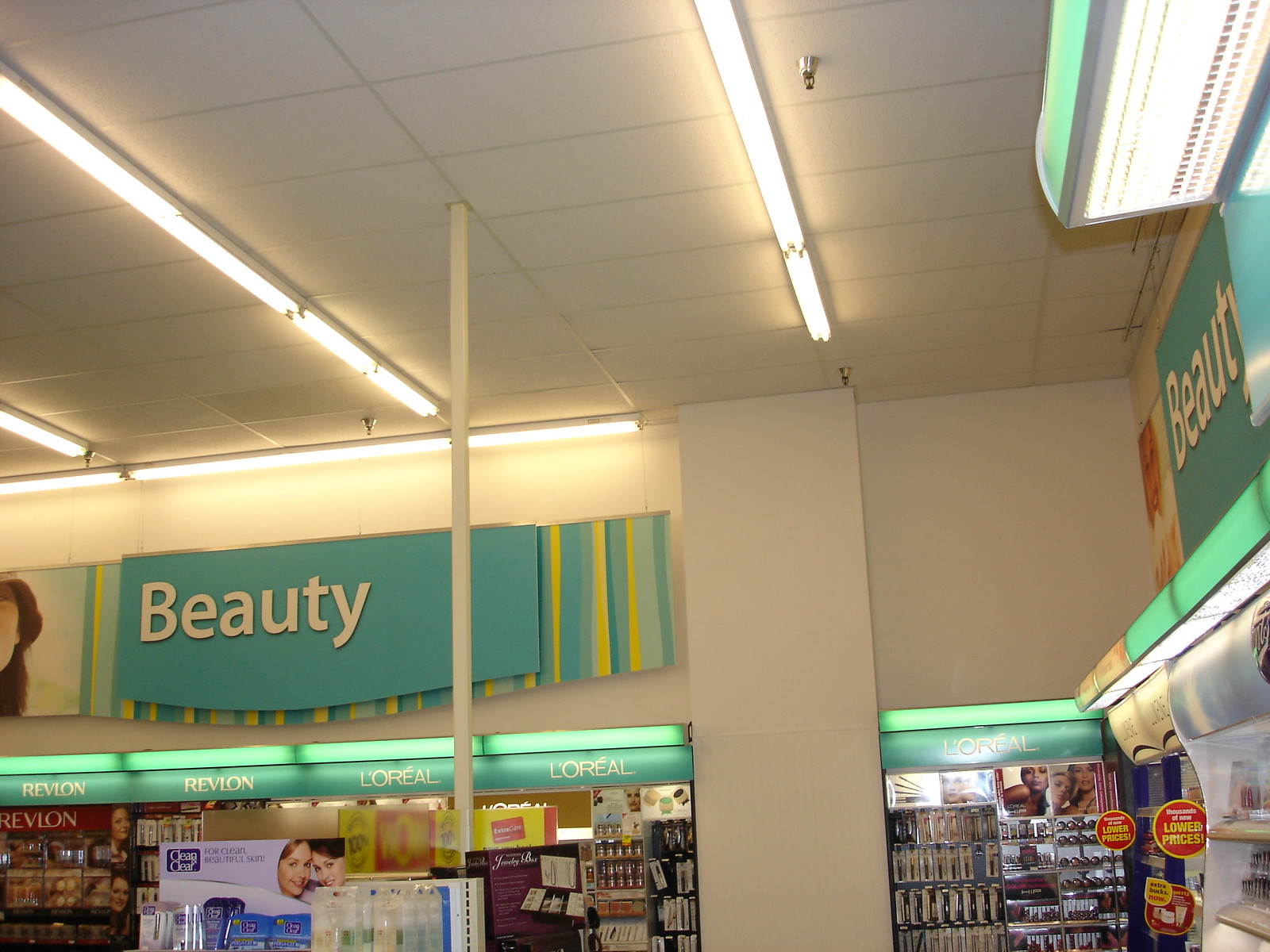This photo appears to have been taken inside the beauty section of a store, which could be part of an indoor mall or a large retail space. The setting is brightly lit by fluorescent lights inset into a ceiling of drop-in tiles, and also features silver sprinklers. Prominently displayed on the pale blue and turquoise walls are large signs that read "Beauty," some of which also feature images of smiling women. These signs are accented with yellow and blue stripes. Below them, illuminated advertisements for well-known makeup brands like L'Oreal and Revlon can be seen, alongside various product stations showcasing items such as makeup brushes and foundations. The walls in this corner section are primarily tan, and there is also signage indicating lowered prices. This detailed layout clearly marks this area as dedicated to beauty and cosmetic supplies.